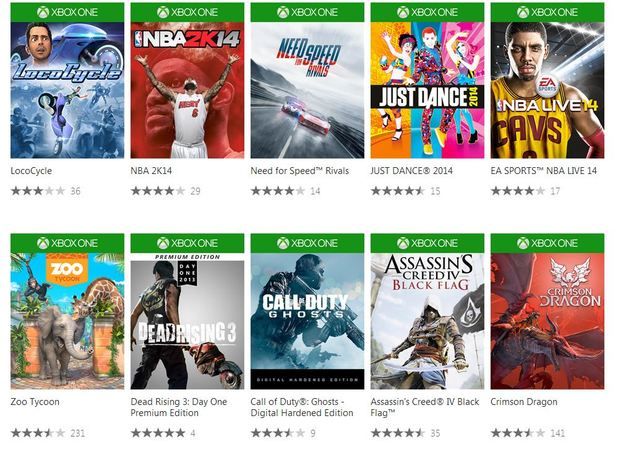The image showcases two neatly arranged rows of Xbox One game cases. In the top row, from left to right, there are five game titles. Each game case features the distinctive Xbox One green banner at the top, followed by an image depicting the game's cover art, and below that, the game's title. Additionally, there's a section for star ratings, indicating the game's reception.

Starting from the left in the top row:
1. "LocoCycle" - The cover art prominently displays a motorcycle, hinting at an action-packed bike game.
2. "NBA 2K14" - Featuring a picture of LeBron James, this game is centered around basketball.
3. "Need for Speed: Rivals" - A high-octane racing game as indicated by its title.
4. "Just Dance 2014" - A vibrant cover suggesting a lively dance game.
5. "EA Sports NBA Live 14" - Another basketball game, displaying a player in a Cavaliers (Cavs) jersey.

In the bottom row, from left to right:
1. "Zoo Tycoon" - The cover features an elephant, giraffe, and monkey, indicating a zoo management simulation game.
2. "Dead Rising 3 Day One Premium Edition" - A survival horror game, part of Capcom's "Dead Rising" series.
3. "Call of Duty: Ghosts Digital Hardened Edition" - A special edition of the popular first-person shooter.
4. "Assassin's Creed" - The cover depicts a hooded character, typical of this historical action-adventure series.
5. "Crimson Dragon" - Featuring mythic creatures, implying a fantasy flight combat game.

Each game case is meticulously organized, making it easy to identify and compare the various titles available for Xbox One.